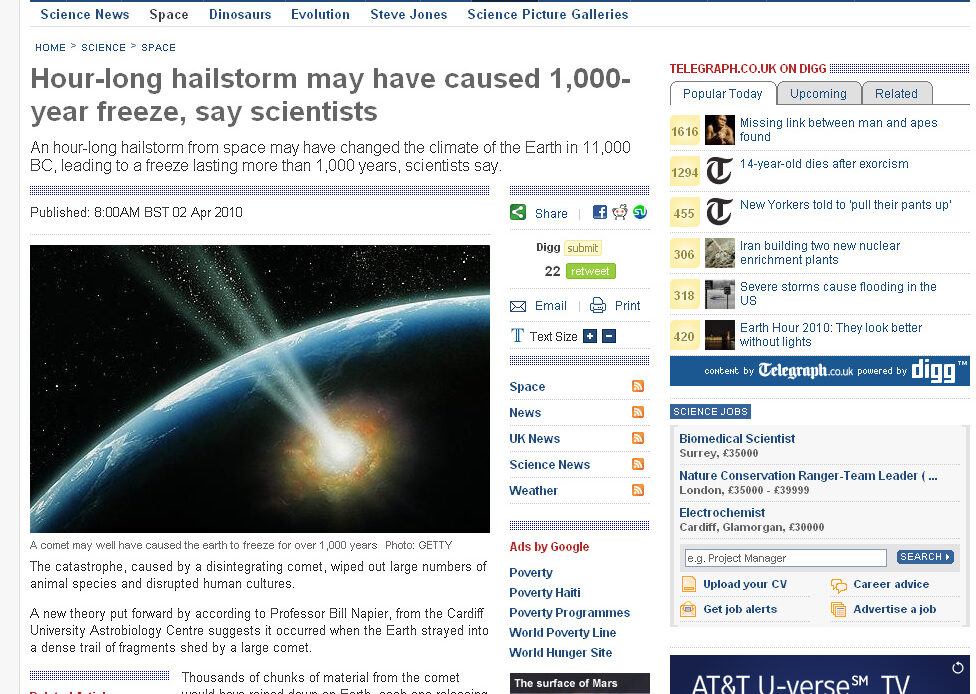The image is a screenshot of a news website displaying an article. At the top of the page, there are various navigation tabs including "Science News," "Space," "Dinosaurs," "Evolution," "Steve Jones," and "Science Picture Galleries." Below the tabs, the category path is listed as "Home > Science > Space."

The title of the article reads: "Hour-long Hailstorm May Have Caused 1,000-Year Freeze, Say Scientists." The subtitle elaborates: "An hour-long hailstorm from space may have changed the climate of the Earth in 11,000 BC, leading to a freeze lasting more than 1,000 years, scientists say."

The publication information specifies that the article was published at 8 a.m. BST on April 2, 2010. To the right of this information, there are share options, including icons for Facebook, Reddit, and another unspecified platform. Further below, additional options for email, printing, and text size adjustments for the editor are available.